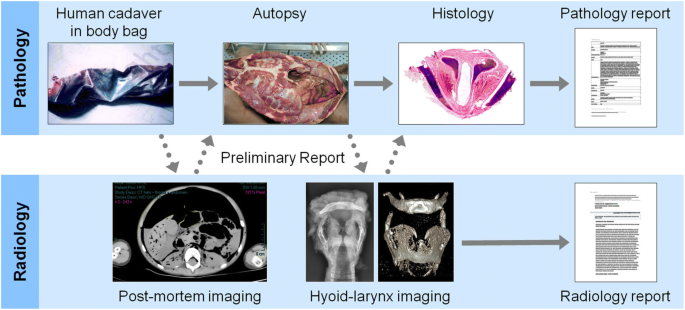This detailed diagram, found in a science textbook, illustrates and contrasts the procedures and processes involved in pathology and radiology for determining the cause of death. The diagram is bifurcated into two main sections, each with a light blue background: the upper section labeled "pathology" to the left, and the lower section labeled "radiology." 

In the pathology section, a series of images and charts is sequenced to show the progression from examining a human cadaver in a body bag, to performing an autopsy where internal parts are visible, followed by histology which zooms in on specific tissues or organs for further analysis, and concluding with the pathology report.

Separating the two sections is a central area labeled "preliminary report." The radiology section beneath this central area includes images of post-mortem imaging, possibly utilizing MRI technology, moving next to detailed imaging of the hyoid larynx, and culminating in the radiology report.

Overall, this rectangle-shaped diagram employs a variety of labeled photographs and charts to encapsulate the flow of an investigation from the discovery of a body to the determination of death through specialized imaging and detailed analysis.